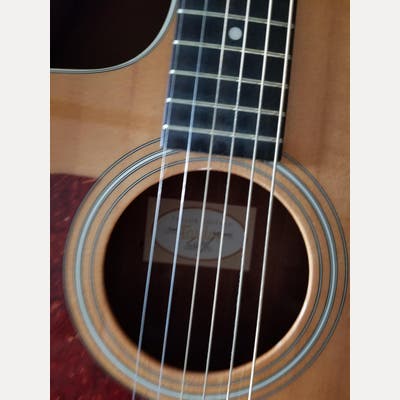This detailed photograph captures a close-up view of an acoustic guitar, specifically highlighting the sound hole and the strings. The guitar features a light wooden finish, with a prominent sound hole in the center where all six strings pass over. Surrounding the sound hole are decorative rings in white and green hues. To the bottom left of the hole, there's a striking red pick guard that adds texture and color contrast to the light brown wooden body. Inside the sound hole, a label with an oval design in white is set against a brown square background, though the text remains illegible due to the image's blurriness. Additionally, a portion of the black neck and frets can be seen, as well as a fragment of a white dot indicating a chord position. Overall, this rectangular, vertically-oriented photo provides a rich, zoomed-in detail of the guitar's central features.